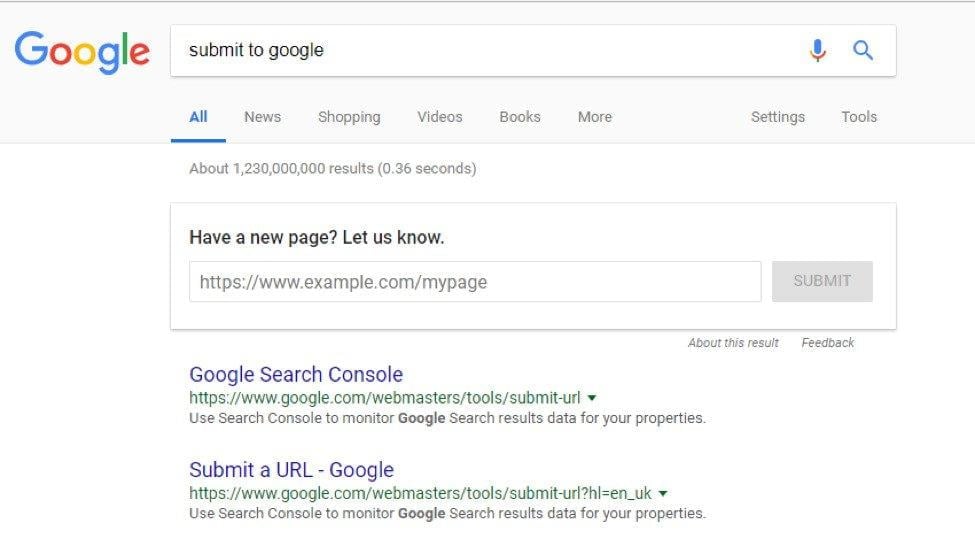This image is a detailed screenshot of the main Google search page. At the very top of the page, there's a search bar containing the text "submit to Google." Directly below the search bar, there are several tabs including "All," "News," "Shopping," "Videos," "Books," with an option for "More" to explore additional search categories. To the right side of these tabs, you can find the "Settings" and "Tools" options.

The screenshot includes familiar icons like a magnifying glass symbolizing the search function and a microphone icon allowing for voice searches. The displayed search results excerpt indicates approximately 1,230,000 results found in 0.36 seconds.

There's also a brief tutorial prompting users with the message, "Have a new page? Let us know," which appears to be a feedback request. Towards the bottom of the screenshot, there's a mention of "Google Search Console by Webmaster Tools," indicating tools available for webmasters. Finally, there's an option to "Submit a URL," suggesting functionalities for submitting URLs to Google's index.